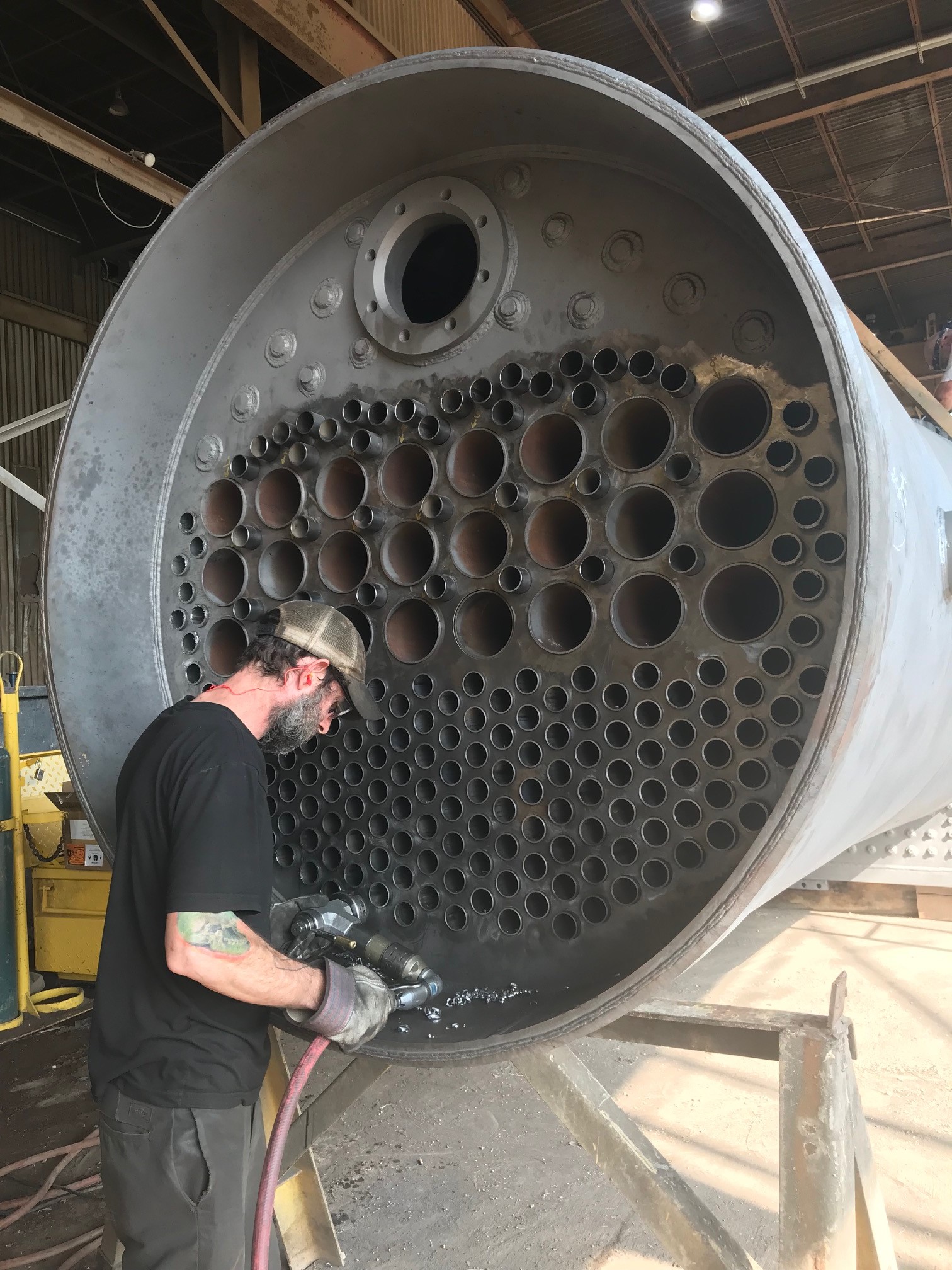The image depicts a large, gray, cylindrical machinery part with a matte finish, positioned horizontally on two sawhorses in a warehouse. The cylindrical object features numerous circular openings of various sizes, starting with smaller ones near the bottom, mid-sized ones progressing upward, and culminating in one large hole near the top end where an end cap with multiple rivets can be seen. 

In front of this mechanical component, a Caucasian man with dark hair and a graying beard is working attentively. He is wearing a black t-shirt, slightly lighter black pants, welding gloves, and safety equipment including a baseball cap, earplugs, safety glasses, and holds an air compressor tool plugged into one of the lower smaller openings. The man has a prominent tattoo on his forearm and is surrounded by metal shavings scattered along the edges of the basin he is working on. The clear focus of the image is the interaction between the man and the complex piece of machinery, indicating a detailed and meticulous engineering process.